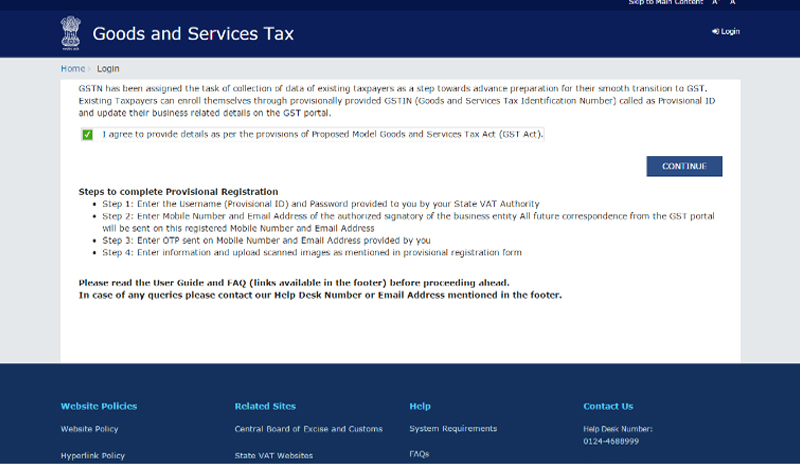The webpage displays a light blue background with a central white box. A navy blue ribbon runs across the top, featuring a white text that says "Goods and Services Tax" alongside a crown-like icon. Below the navy blue ribbon, the webpage showcases "Home" in bright blue and "Login" in gray text within the light blue background. 

Inside the white box, the text explains that GSTN has been tasked with collecting data from existing taxpayers to facilitate a smooth transition to GST. It details that existing taxpayers can enroll using their provisionally provided GSTIN (Goods and Services Tax Identification Number) and update their business information on the GST portal.

A white ribbon with a green checkmark follows, accompanied by the text, "I agree to provide details as per the provisions of the proposed model Goods and Services Tax Act (GST Act)." Finally, a navy blue button labeled "Continue" in white text is positioned to the right below this validation ribbon.